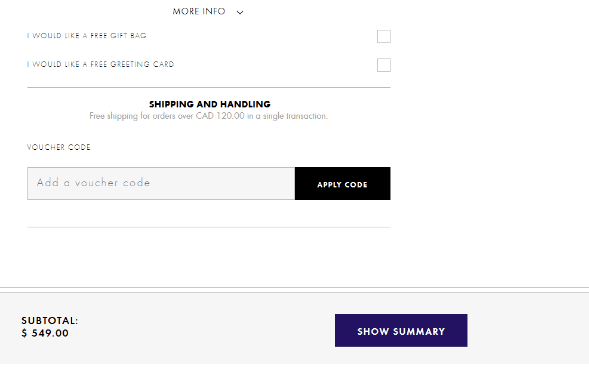The screenshot captures a section of someone's online shopping basket, indicating a substantial total amount of $549. Though the specific items in the basket are not visible, the high cost of the selected merchandise is noted. Adjacent to this total, there is a purple option labeled "Show Summary" for further details. Above the total, a text box is displayed where users can input a discount or promotional code; however, this particular user has decided not to use a code, opting to purchase the items at full price. 

Additional options are listed above, offering the selection of a free greeting card and a free gift bag. Both of these options remain unchecked by the user. A message from the brand informs customers that free shipping and handling are available for orders exceeding CAD 120 in a single transaction, implying that the user's order qualifies for complimentary shipping.